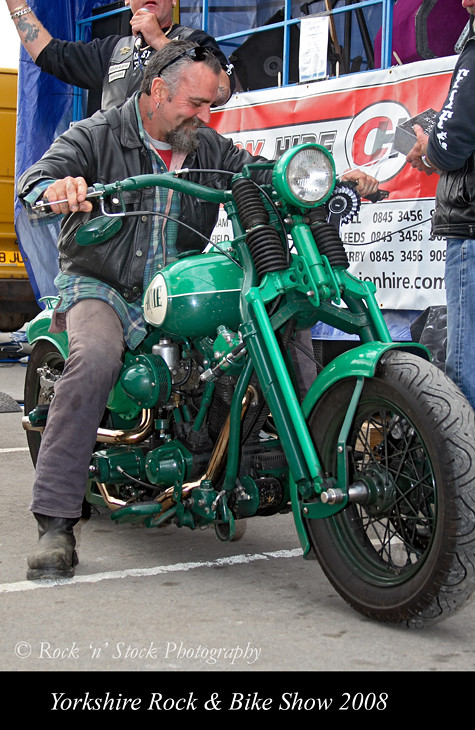The image depicts a bearded man smiling down while seated on a vintage green motorcycle, which features a green gas tank, green carburetor, green handlebars, and black springs around the front headlight. The man, clad in a black leather jacket, a green and white checkered shirt over a white shirt, and black jeans with a stain at the knee, wears black motorcycle boots and has sunglasses resting on top of his head. In the background, indicative of the Yorkshire Rock and Bike Show 2008, a person, wearing a black vest, short sleeves, and bracelets, can be seen with a microphone and displaying tattoos. There's a red banner with unreadable numbers behind them, further setting the scene of the event, which is confirmed by the "Yorkshire Rock and Bike Show 2008" and "Rock and Stock Photography" text at the bottom of the image.